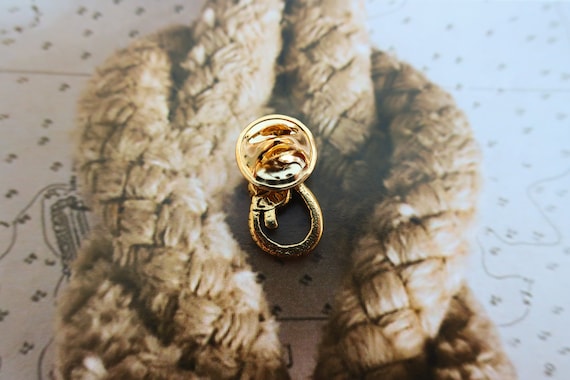The image prominently features a gold-plated lapel pin, centrally positioned against a background of a beige, tightly woven rope tied in a bowline knot. The lapel pin, which is almost circular with a concave design, features a hook, clasp, and ring-like structure at the top and displays an inscription in its middle. The rope is brown and laid out on a white tiled surface, which has speckles that resemble a nautical map. The setting and style evoke a sense of nautical or marine activity, and the pin itself likely symbolizes sailing, making it suitable for a formal outfit in related contexts.